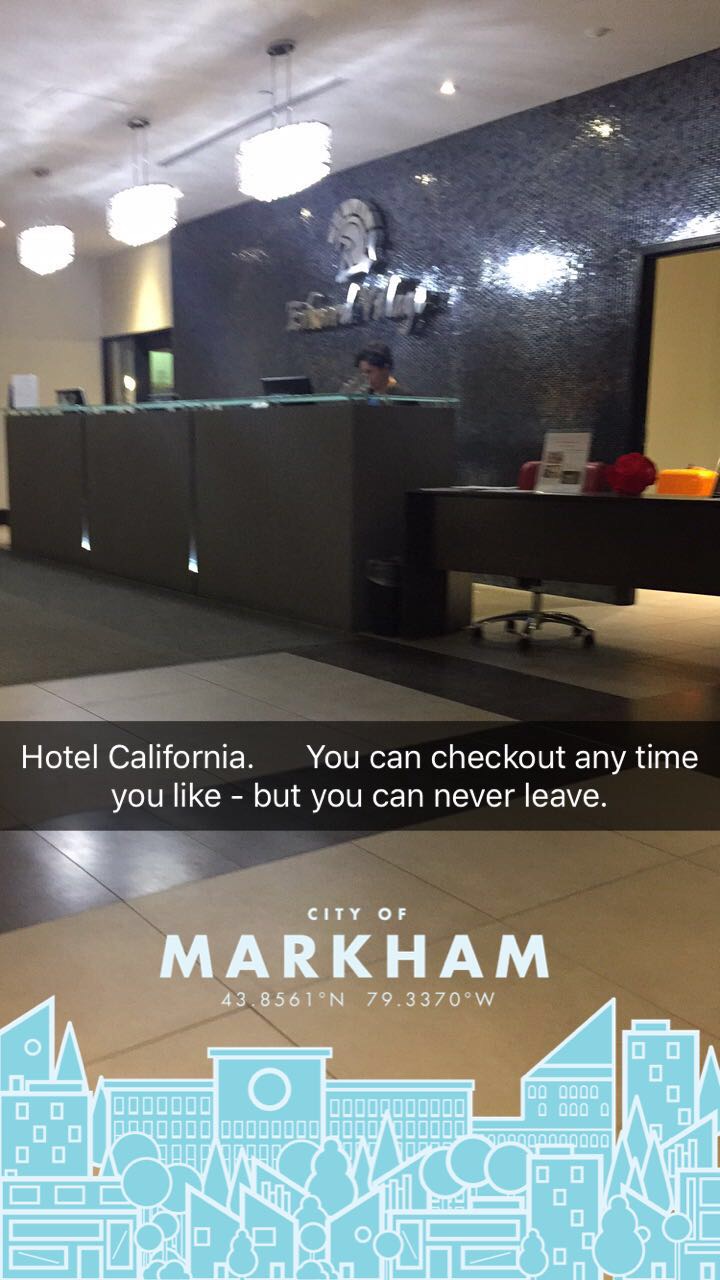This is an image of a hotel lobby, possibly named something with the word "village" in its title. Centered on a shiny, crinkly blue backdrop with varying blue shades, there's a silver text partially obscured but featuring a logo resembling a knight’s or Roman gladiator’s head. Prominently displayed is a banner that reads, "Hotel California. You can check out anytime you like, but you can never leave," with "City of Markham" written underneath in white letters, followed by geographic coordinates: 43.8561°N, 79.3370°W. Below this, there is a pencil-style drawing of a village in light blue and white, showing houses and trees.

The lobby features three reception desks, and at one of them sits a person with black hair working at a computer. To the right, there's a concierge desk adorned with red flowers and a card holder providing information. Additional details include a large entryway, overhead chandeliers, and sets of fluorescent lights casting a well-lit ambiance over the gray, dark gray, light gray, and light orange or tan tiled floor, all contributing to a visually rich and detailed setting.